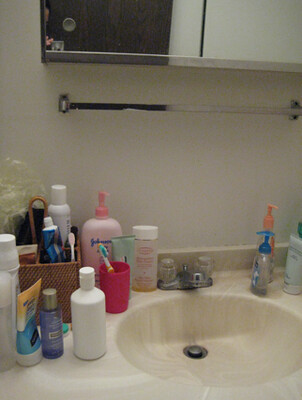The bathroom sink countertop is pristine white, though the sink itself is marred by noticeable brown dirt. The faucet is a sleek silver design with two clear handles. Above the sink, a silver bar is installed, and further up, a medicine cabinet with a mirror occupies the wall. The countertop is cluttered with various items: on the right-hand side, there is a soap dispenser and a clear bottle with a blue pump lid. A brown basket holds toothpaste and other spray bottles, while a pink cup contains a toothbrush. Behind the cup, there is a large, pink Johnson & Johnson pump-action bottle. The sink’s drain is positioned upward, and in the corner of the mirror, part of a person's reflection is visible.